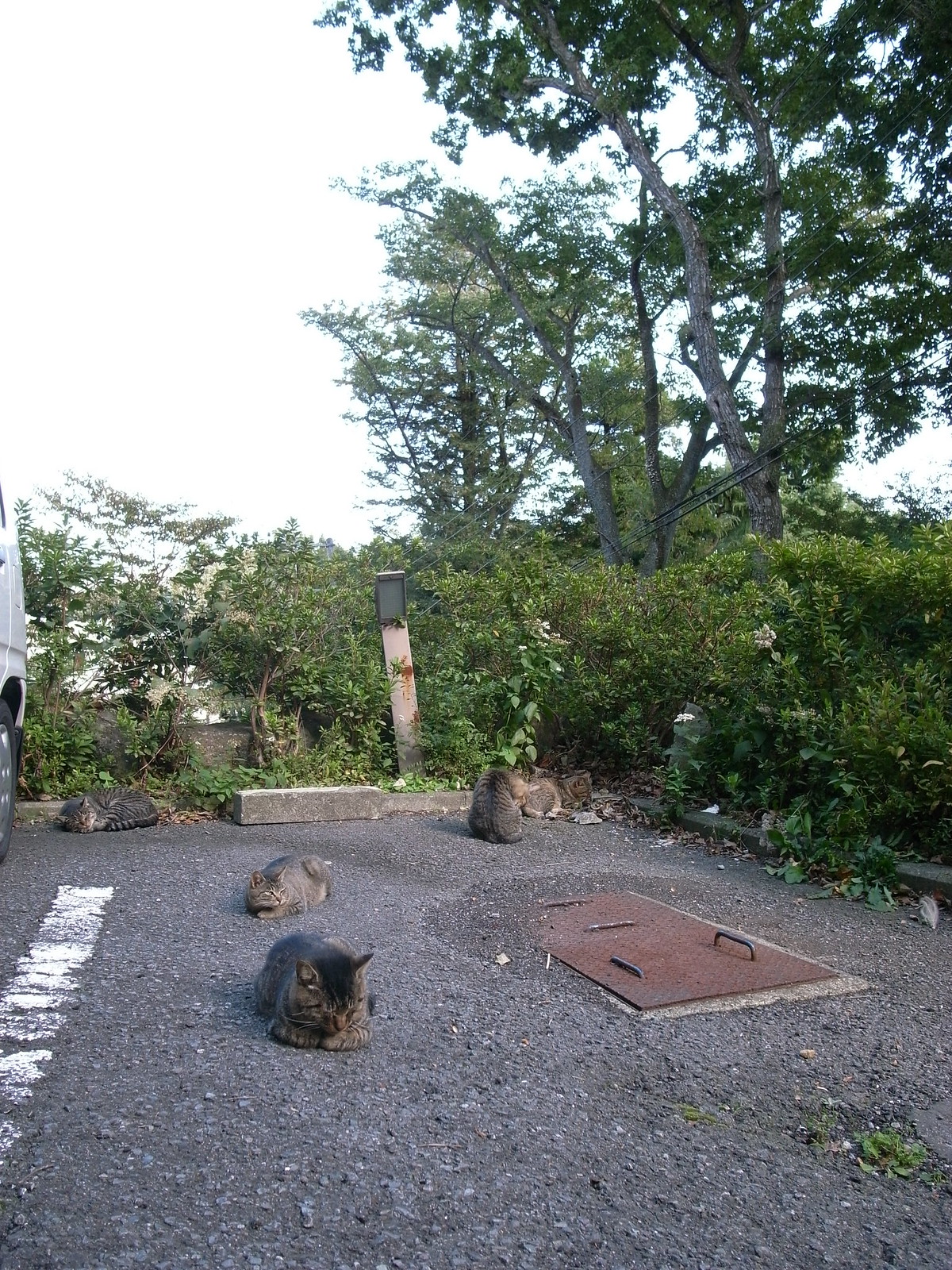In this photograph, we observe a tranquil scene nestled in the corner of a parking lot. The focal point is an empty parking stall, characterized by its gravelly asphalt and marked by a faint white parking stripe in the lower left corner. A glimpse of a van is also visible, stationed in the adjacent spot, with green hedges forming a natural boundary in the background. Amidst this urban setting, four gray and black striped tabby cats lounge contentedly, their paws tucked neatly beneath them in classic "cat loaf" positions. One cat is prominently in the foreground, while the others are slightly further back. Their arrangement, with one possibly licking its paws, conveys a sense of restful camaraderie.

The parking area is accentuated by a mix of flora, including rose bushes with blooming flowers and tall, leafy trees that reach the upper frame of the image. A rusty, heavy metal trap door is conspicuously set into the ground, adding an industrial element to the scene. The composition suggests that there's possibly more feline company lurking within the hedges, hinting at the hidden depths of this peaceful enclave. Overall, the image captures a moment of calm and natural beauty amid the everyday functionality of a parking lot.